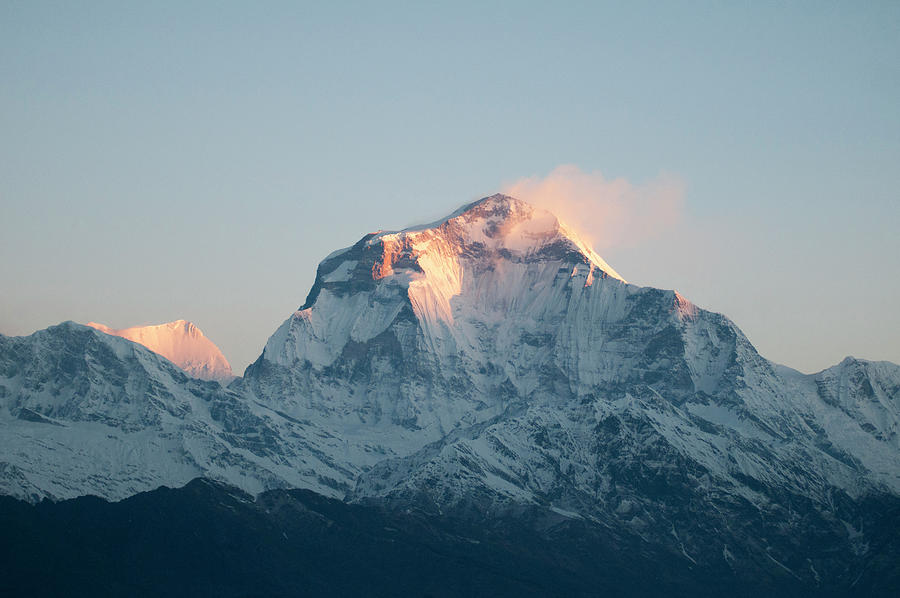This breathtaking photograph captures a jagged, snow-covered mountain range under a light blue-grey sky. The centerpiece is a prominent peak that aligns with a thin band of clouds, its apex bathed in a warm, orange hue from the rising or setting sun. The snow appears light, with rocky protrusions visible even in the most covered areas. Flanking this central peak are two lesser, snow-covered summits; the one on the left is fully illuminated by the sunlight, while the one on the right remains cloaked in shadow. The lower regions of the mountains cast dark shadows, with some areas possibly showing dark green foliage, adding depth and contrast to the scene. Wisps of fog or smoke drift up from the central peak, enhancing the dramatic and serene atmosphere of this majestic landscape.